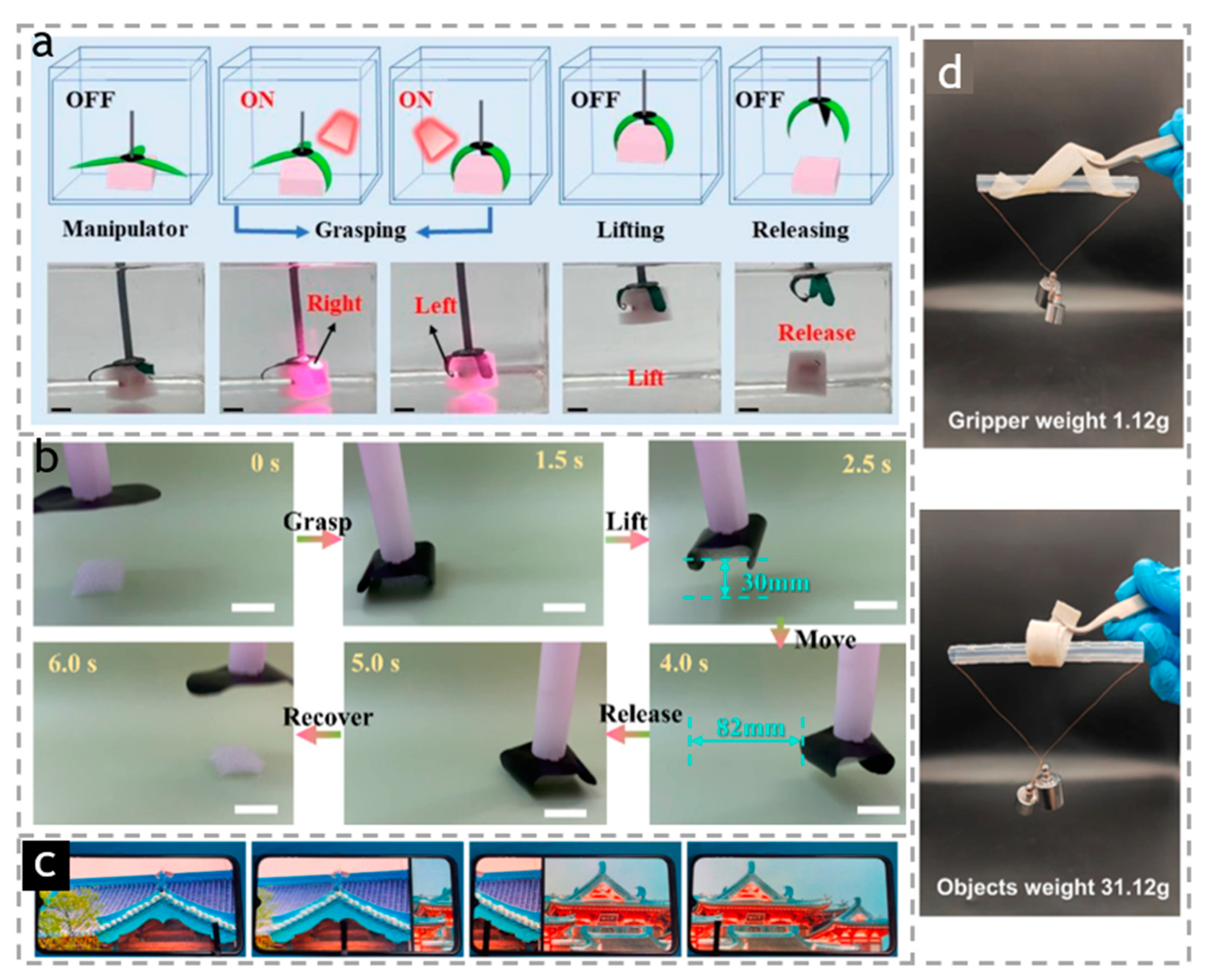The image is a detailed, full-color schematic with multiple sections demonstrating the functions and specifications of a mechanical gripper device. The overall image is square, bordered by a light gray dashed line. 

In the upper left corner, labeled with a small letter 'A', there is a blue rectangle containing five blue squares in a grid. The first and last squares are labeled "off," while the middle three are labeled "on," depicting the positions of a switch that controls the device, resembling a crane-like mechanism. Below this section is a color version of the same grid with visual depictions of the gripper's actions, including moving left and right, lifting, releasing, grasping, and repositioning objects.

To the right, labeled 'B', is a series of six images of a purple stick with a black base, possibly illustrating different stages or components of the device. Below these are five images representing colored Chinese buildings, which might be unrelated decorative elements.

The bottom part of the image includes a timeline with green segments marked with specific time intervals: 0 seconds, 1.5 seconds, 2.5 seconds, 6.0 seconds, 5.0 seconds, and 4.0 seconds. This likely indicates the operation or cycle times of the gripper. The background here is blue, showing what appears to be the roof of a structure or a section of a machine frame.

On the right side of the image, there are two key measurements: the first states "gripper weight: 1.12 grams" and the second "object's weight: 31.12 grams," reflecting the capacity and precision of the device. Additionally, there is an image of a person manipulating the gripper using forceps while wearing blue surgical gloves, hinting at a possible application in a precise or sterile environment.